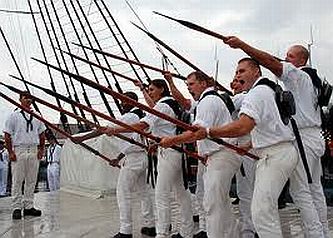The image depicts a small, rectangular, low-resolution photograph of what appears to be a group of cadets or sailors engaged in a training exercise, outdoors during the daytime. The sky is a mix of gray and white, indicating overcast weather. On the right side of the image, there are at least six young men arranged in two rows—four in the front and three behind—clad in white shirts and pants with black shoes and backpacks. Their apparent ethnicities include Hispanic, white, and possibly black. Each of these men is holding a long, pointed object resembling a spar, pole, or possibly a pool cue. Some wear old-style 19th-century sailor hats, resembling shallow cylinders atop wide brims, and appear to be shouting as they point their spars from right to left.

In the bottom left corner, another man dressed similarly in a white shirt and off-white pants stands with his hat, secured by a knot, hanging from his back. He is positioned with his arms at his sides, attentive but unarmed. Behind the group, in the upper left corner of the image, the rigging and ropes of a tall ship are visible, suggesting that the platform they stand on might be the deck of a ship. Despite the blurriness, the image vividly captures a moment of disciplined drill or demonstration, underscored by the formal attire and coordinated action of the participants.